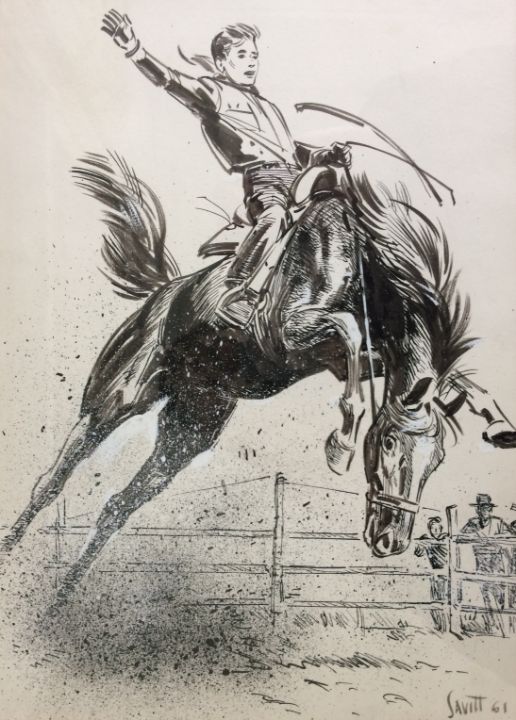The image is an old black-and-white illustration of a dramatic rodeo scene, capturing the intensity and action with exquisite detail. The central focus is a wild-eyed, dark horse with a dark mane and tail, contrasted by a striking white blaze running down its forehead to its nose. The horse is bucking high into the air, its powerful front legs thrusting forward while its back legs kick up, sending dust and dirt flying around its hindquarters. 

A man is seated on the horse, gripping the reins tightly with his left hand while his right hand is raised high in the air. He is dressed with a scarf around his neck and appears to be wearing gloves, notably missing a hat. 

In the background, a wooden gate stands, behind which a couple of spectators observe the action. One of the onlookers is taller and wears a hat, while the other is shorter and hatless. The illustration is signed "Savitt, S-A-V-I-T-T, 61" in the bottom right corner, adding an element of authenticity and historical context to the artwork.